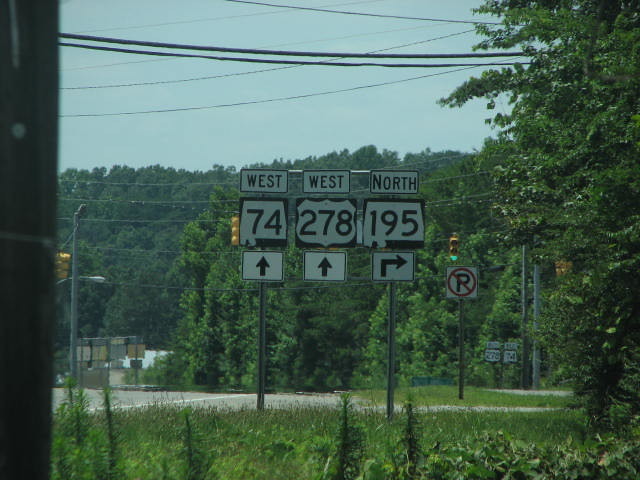This photograph features three prominent street signs indicating highways, positioned alongside a road bordered by lush greenery. The first sign on the left, square in design and in black and white, directs travelers straight ahead for West 74, denoted by an upward arrow. The middle sign, styled with a distinctive sheriff's deputy badge shape, guides drivers straight ahead for West 278, also marked with an upward arrow. The final sign on the right, another square sign in black and white, instructs motorists to turn right for North 195. The setting is a rural area with ample trees and grass surrounding the signs, creating a peaceful, countryside ambiance. A stoplight situated off to the left adds to the roadside infrastructure, while the absence of cars emphasizes the tranquil, almost deserted appearance of the scene.